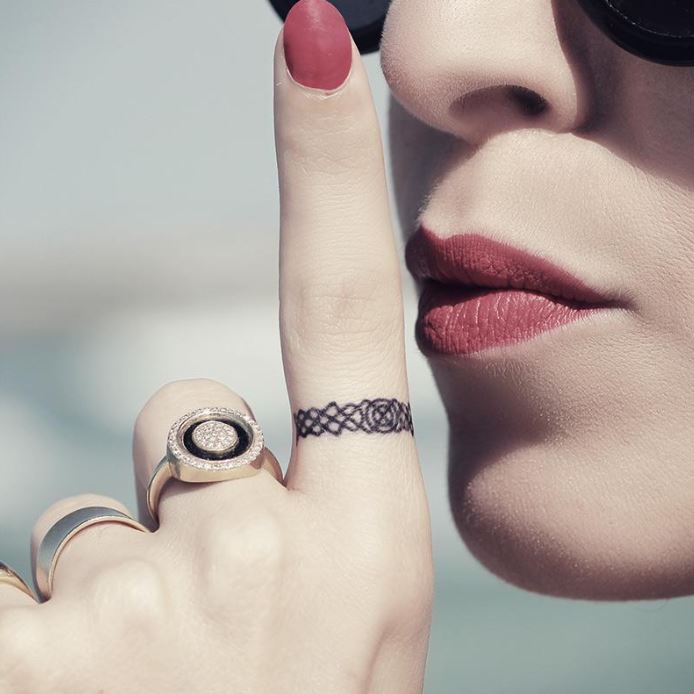This is a close-up photograph of a fashion art piece featuring part of a woman’s face and hand. The woman, possibly of European descent, has smooth, pale white skin and wears bright red lipstick. Only the bottom left side of her face is visible, revealing the tip of her nose, the side of her mouth, and the bottom half of her black sunglasses. Her lips are closed and puckered forward.

The woman’s left hand is held up in front of her lips in a 'be quiet' gesture, with her index finger raised. She has matching red nail polish on her fingers. At the base of her index finger is a tattoo resembling an interlacing design of braided black lines with a circle in the middle, giving the appearance of a ring. In addition to the tattoo, she is wearing three golden rings: one on her middle finger featuring diamonds set in a black circle, and simpler rings on her ring finger and pinky, which extends out of the frame.